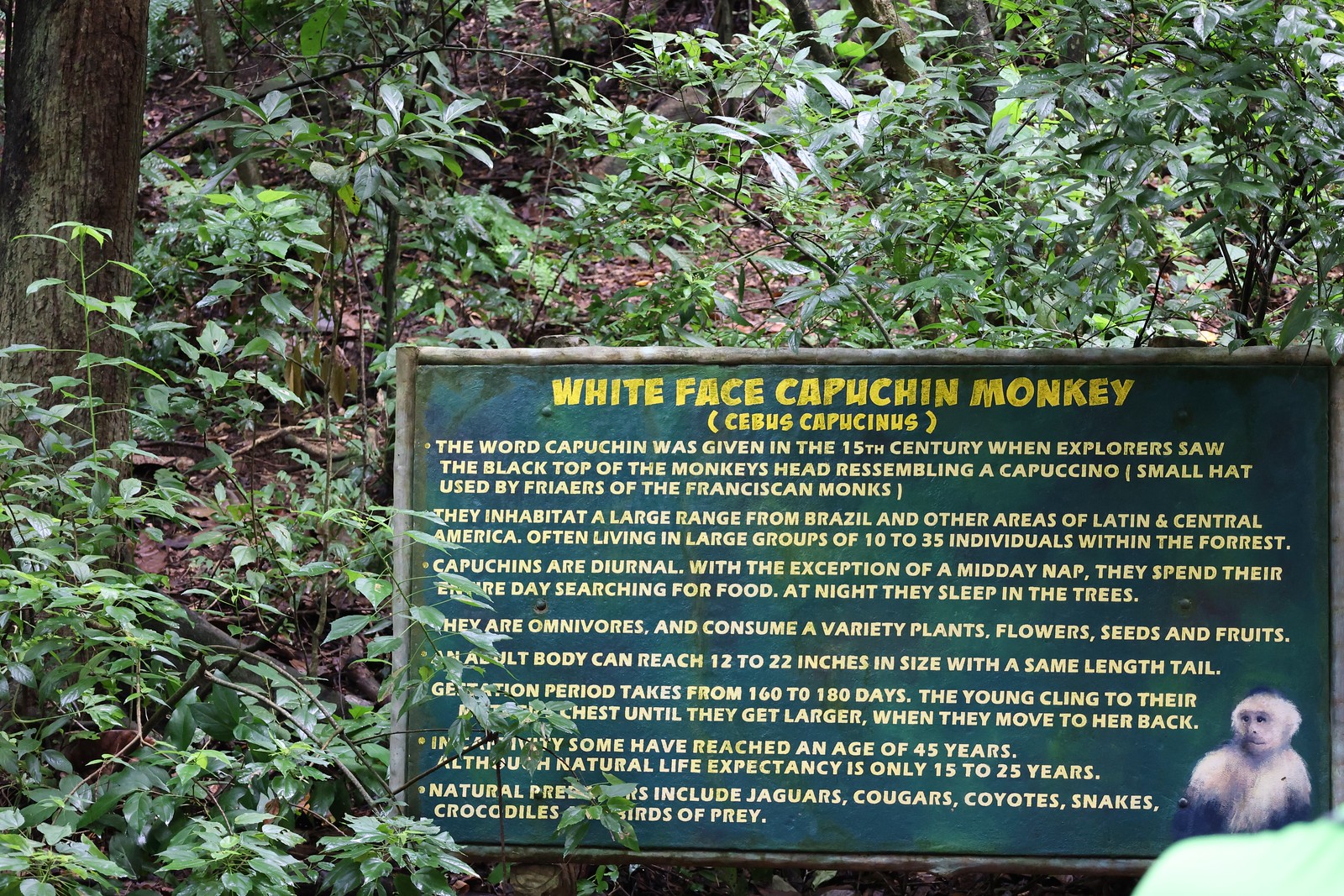The image depicts a detailed outdoor scene resembling a lush forest or jungle. In the upper left, a prominent tree trunk stands amidst dense, verdant foliage composed of numerous small plants. The setting, bathed in daylight, showcases various shades of green, yellow, brown, tan, black, white, and gray.

In the bottom right corner, partially nestled among the bushes and trees, is a rectangular placard with a wooden border. The sign, primarily black with vibrant yellow lettering, announces in large, all-caps text: "WHITE-FACED CAPUCHIN MONKEY," followed by its Latin scientific name in parentheses below. Slightly lighter yellow bullet points detail the monkey's habitat and behavior, noting that they can live between 12 to 25 years but occasionally reach up to 45 years. The Capuchin monkeys are omnivorous, consuming a broad range of plants, flowers, seeds, and fruits. They are social animals, often found in groups ranging from 10 to 35 individuals, inhabiting regions from Brazil through Central America. The monkeys are diurnal, spending their days actively foraging for food and taking a midday nap, and their nights sleeping in the trees. Furthermore, a small illustrated image of a monkey appears on the placard, adding a visual cue to the comprehensive text.